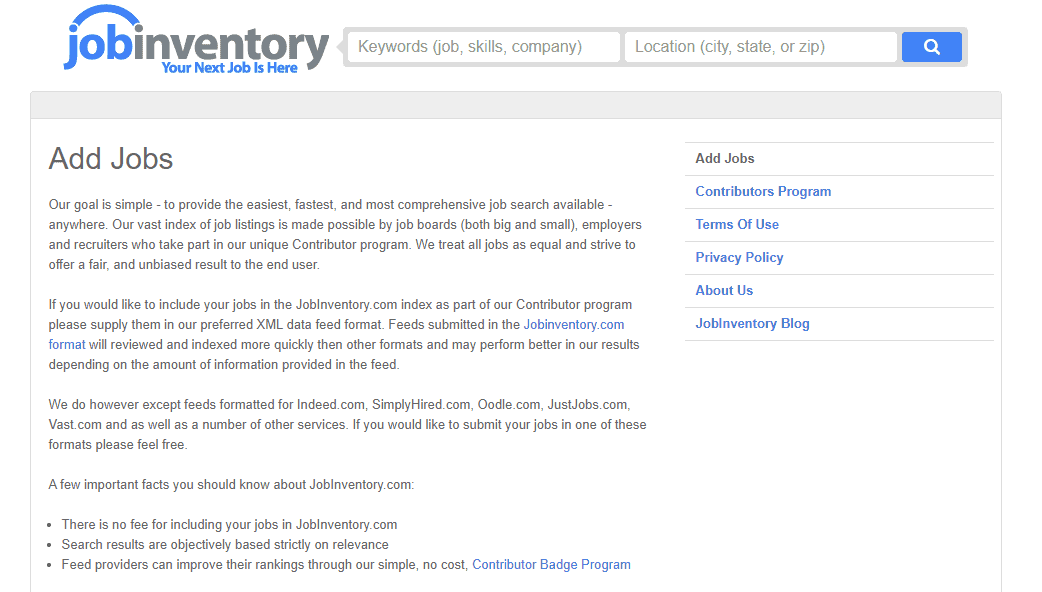Here is the cleaned-up, detailed caption for the image:

---

This image depicts an employment website called "Job Inventory." At the top of the page, the site name is displayed, with "Job" in blue text and "Inventory" in gray text. Below the site name, a prominent blue text headline reads, "Your next job is here." Positioned to the right of this headline are two rectangular search categories. The first box is designated for keyword-based searches, allowing users to input job titles, skills, or company names. The second box facilitates location-based searches, where users can enter city, state, or ZIP code information.

Further down the page, a section labeled "Add Jobs" is displayed. This section includes text that outlines the website's mission: "Our goal is simple: to provide the easiest, fastest, and most comprehensive job search available anywhere. Our vast index of job listings is made possible by job boards, both big and small, employers, and recruiters who take part in our unique contributor program. We treat all jobs as equal and strive to offer a fair and unbiased result to the end user."

The text continues to explain the process for including jobs in the JobInventory.com index as part of the contributor program. Employers are encouraged to submit job listings in the preferred XML data feed format, with a note that feeds submitted in this format are viewed and indexed more quickly and may perform better in search results, depending on the information provided. Additionally, the website accepts feeds formatted for other job listing services such as Indeed.com, SimplyHired.com, Google.com, JustJobs.com, and Fast.com.

On the right side of the page, a list of categories appears, all in blue text except for the first one. The categories listed are: "Add Jobs and Contributors Program," "Terms of Use," "Privacy Policy," "About Us," and "Job Inventory Blog."

---

This caption provides a clear and detailed description of the content and layout of the employment website presented in the image.